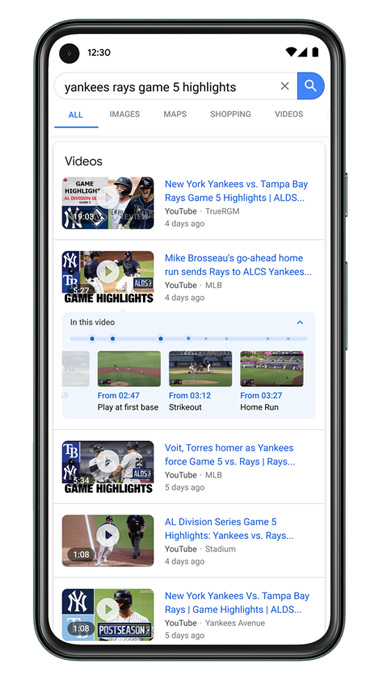This detailed caption describes a screenshot framed within a digital image of a silver cell phone. The phone's borders feature two buttons on the right side: a smaller top button and a larger bottom button. The screenshot itself displays various elements within the simulated phone screen.

In the upper-left corner of the screenshot, the time is displayed as 12:30, and the upper-right corner shows a fully charged battery icon. Directly below is a search bar with the query "Yankees Raise Game 5 Highlights." Beneath the search bar, there are navigational options: "All," "Images," "Maps," "Shopping," and "Videos," with "All" highlighted in blue and underlined.

The following two rows are dedicated to video results. Each result features a video thumbnail on the left, marked with a triangle play icon. To the right of the first thumbnail, text reads "New York Yankees versus Tampa Bay Rays Game 5 Highlights ALDS YouTube," followed by "four days ago" in blue, indicating a live link. The next video result mirrors this format, with a thumbnail on the left and the text "Mike Brousseau's Go Ahead Home Run sends Rays to ALCS Yankees four days ago on YouTube" on the right. 

Underneath the second video description is a light blue section displaying a menu of video chapters, titled "In this video." It lists chapters such as "from 2:47 play at first base," "from 3:12 strikeout," and "from 3:27 home run," all in blue as clickable live links. In the bottom-right corner of this section is an upward arrow, serving as an expand button to show more chapter highlights if clicked.

The backdrop of the entire screenshot is a clean white background, with highlighted sections in light blue to distinguish interactive elements.